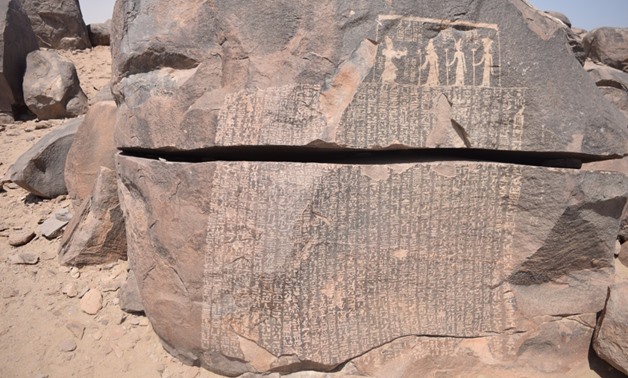This is a color, landscape-oriented photograph depicting a large, gray boulder split horizontally across the middle, revealing Egyptian hieroglyphics engraved on both the upper and lower sections, where the split occurs. The central feature of the engraving is a panel towards the top right, showcasing four Egyptian figures in profile, holding staffs, separated by rectangular borders. The characters and figures reveal an inner portion of the stone that is light pink, contrasting with the dark gray surface. Surrounding this boulder are smaller rocks and fine, light brown and pinkish dirt, set against a background that hints at a blue sky, suggesting a desert environment, potentially in Egypt. This intricate stone engraving resembles the Famine Stela, a notable piece of Pharaonic diary. The photograph captures the scene in a detailed, realistic style, emphasizing the extraordinary and enigmatic presence of these ancient carvings in an otherwise ordinary rocky landscape.